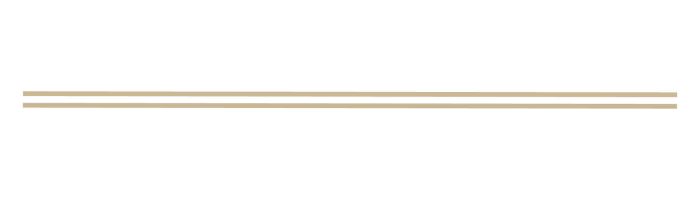The image features two long, parallel horizontal lines extending from the left to the right side against a plain white background with no visible borders. Both lines are straight and evenly spaced, with a narrow strip of white separating them. Each line is approximately an eighth of an inch in width, and the gap between them is around the same size. The lines are light tannish brown or beige in color, creating a stark contrast against the white background. The overall composition is minimalistic, consisting solely of these two identical horizontal lines with no other text or objects present. The simplicity and uniformity dominate the visual, making it an image of two straight, parallel lines on a solid white backdrop.